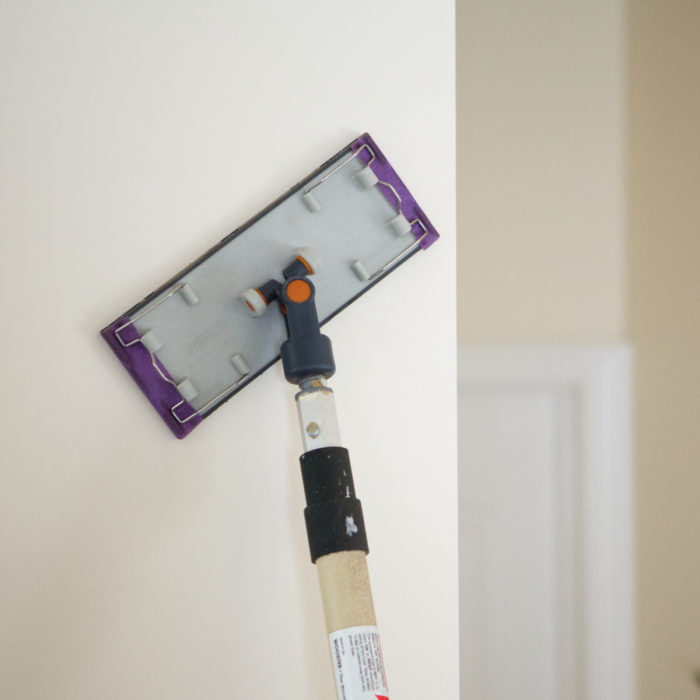The photograph presents a carefully composed interior scene with a distinct color gradient and specific objects subtly placed within the frame. On the left side, a wall painted in a soft lavender hue transitions gradually to an almost white shade towards the center-right of the image, showcasing an elegant color gradient. The right side of the image features another wall, this one a gentle beige. Just off-center, there's the faint outline of a picture frame, presented in a very light gray. The frame is only partially visible, showing just the upper right corner, with what seems to be a large white mat suggesting that any photograph or artwork it might contain is not visible.

To the far left, a metal object is noted. This object is a rectangular device with gray sides and purple ends, featuring a handle. The handle itself is primarily light brown with black accents and attaches to the device at a black joint, highlighted by a small orange dot. The nature of this device suggests it could potentially be a cleaning implement. The overall composition of the photograph is minimalist yet thoughtful, emphasizing the play of soft colors and subtle details.